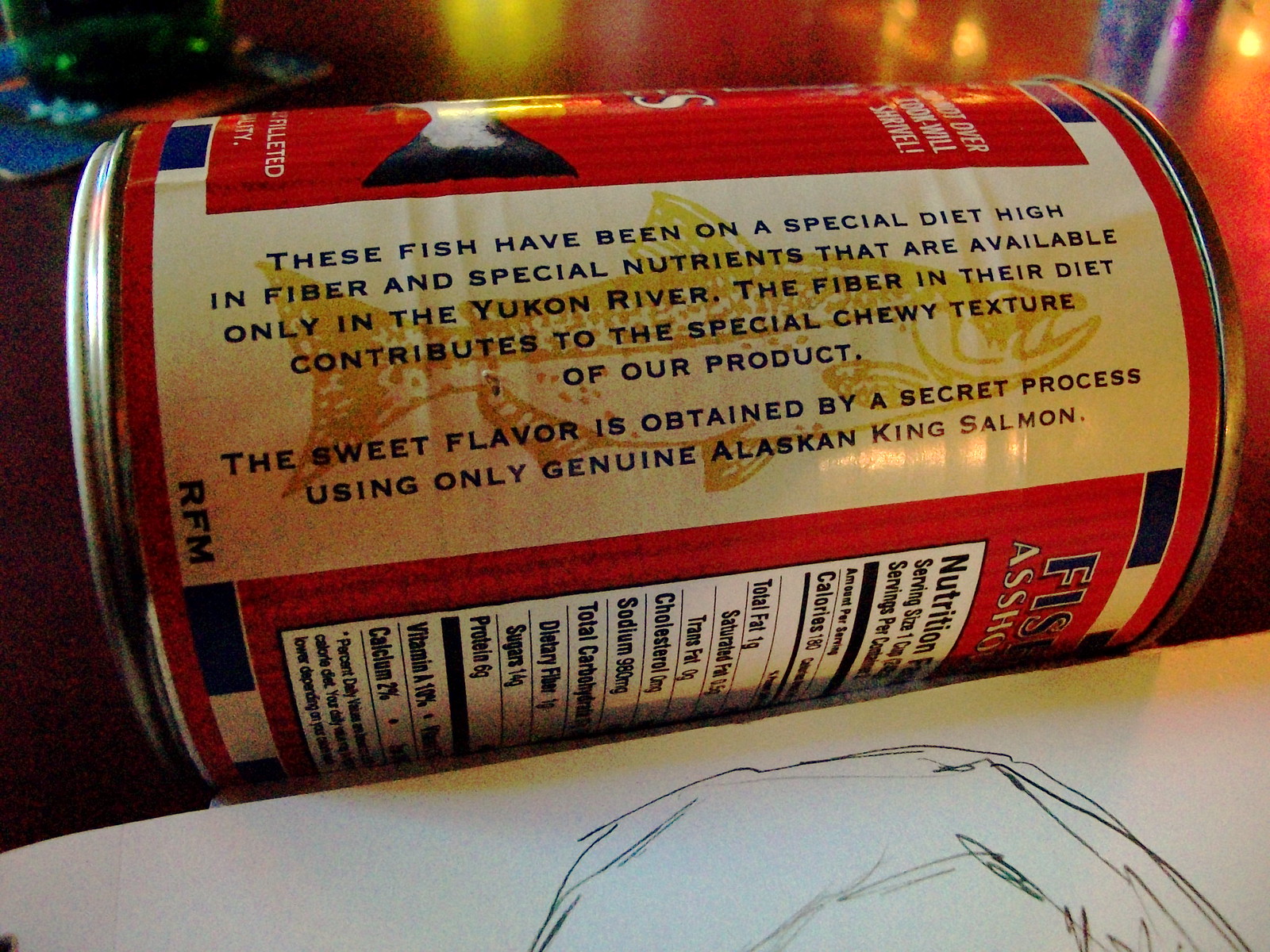This image features the side of a can, which appears to be a food item, likely canned fish, given the prominent fish imagery. The can has a distinctive design with a primarily red backdrop accented by white elements. There is an illustration of a fish, possibly a salmon, indicating the type of fish contained within. The image also includes a white sheet of paper with partial pen drawings, slightly obscured. Adding to the can’s label design, there is blue print on the white background, accompanied by a yellow fish icon. The text reads: "These fish have been on a special diet high in fiber and unique nutrients only found in the Yukon River. The fiber in their diet contributes to the distinctive chewy texture of our product. This sweet flavor is derived from a secret process using only genuine Alaskan King Salmon."